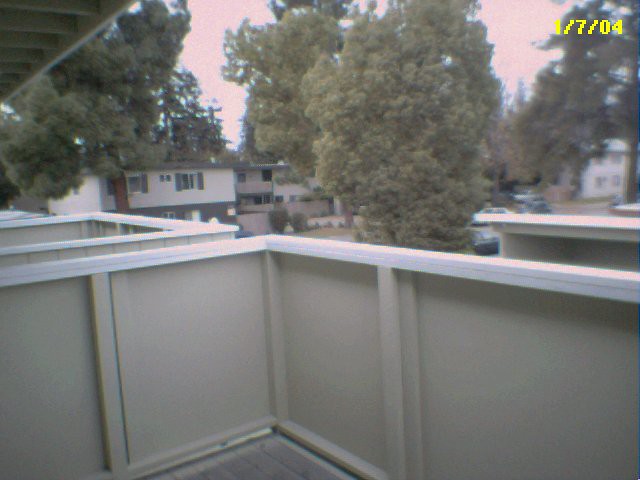A photograph captured from a balcony of what appears to be an apartment complex. The balcony features a wooden floor and waist-high tan-colored walls on both sides, with a white railing encircling the perimeter. Adjacent balconies are visible, spaced a few feet apart. The scene overlooks a residential street, where several green trees provide a lush backdrop. On the street below, two cars—one white and one black—are parked. Directly across the street stands a two-level house, with a gray lower level and a white upper level. In the upper right-hand corner of the image, a yellow date stamp reads "1-7-04".